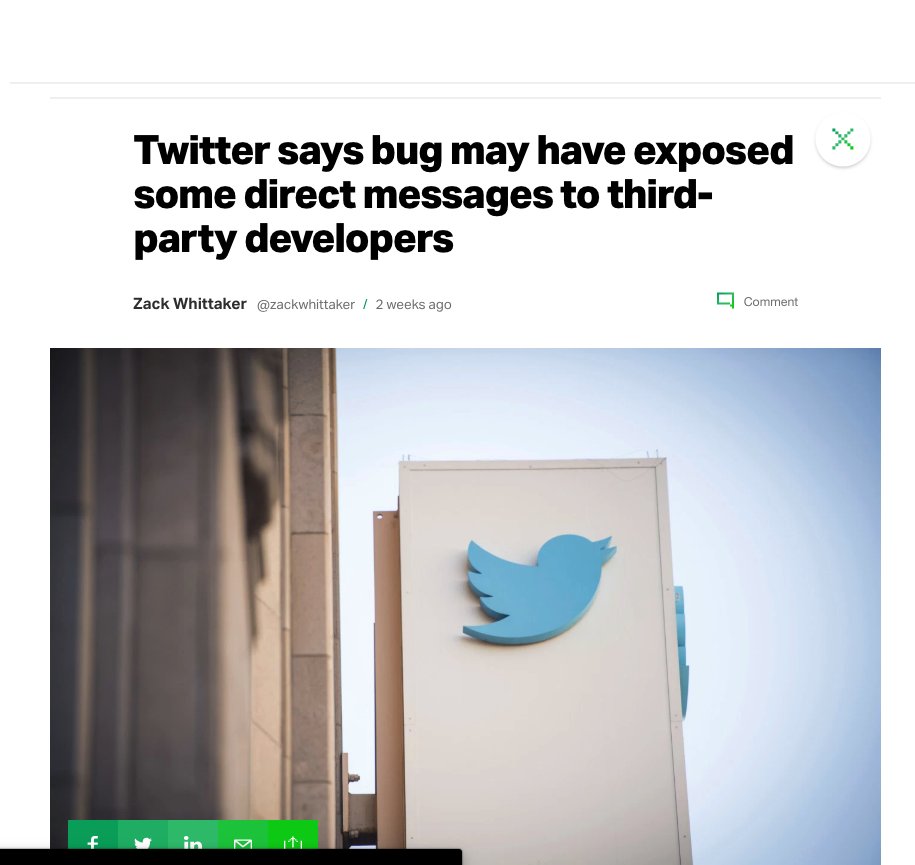Screenshot of a news article headline on a website. The bold header reads, "Twitter says bug may have exposed some direct messages to third-party developers." In the upper right-hand corner, there is a white circle with a dotted X indicating the option to close the notification. The article, written by Zach Whitaker, shows the author's name in bold with the handle "@zachwhitaker" followed by "two weeks ago."

Next to this, a blue speech bubble icon representing comments is positioned to the left of the word "comment," both located on the right side of the header. Below this text, there is an image displaying the iconic Twitter bird in 3D, affixed to the front of a building, functioning like a sign. The facade of the building is partly visible and slightly blurred due to depth of field.

In the lower left part of the image, several social media icons are displayed: Facebook, Twitter, Indeed, and an email icon. Additionally, there is a partially visible share icon inside a small black rectangle, cut off at the bottom of the screenshot. It appears the main content was clipped from the news website, emphasizing the Twitter bird on a building and the related social media sharing options.